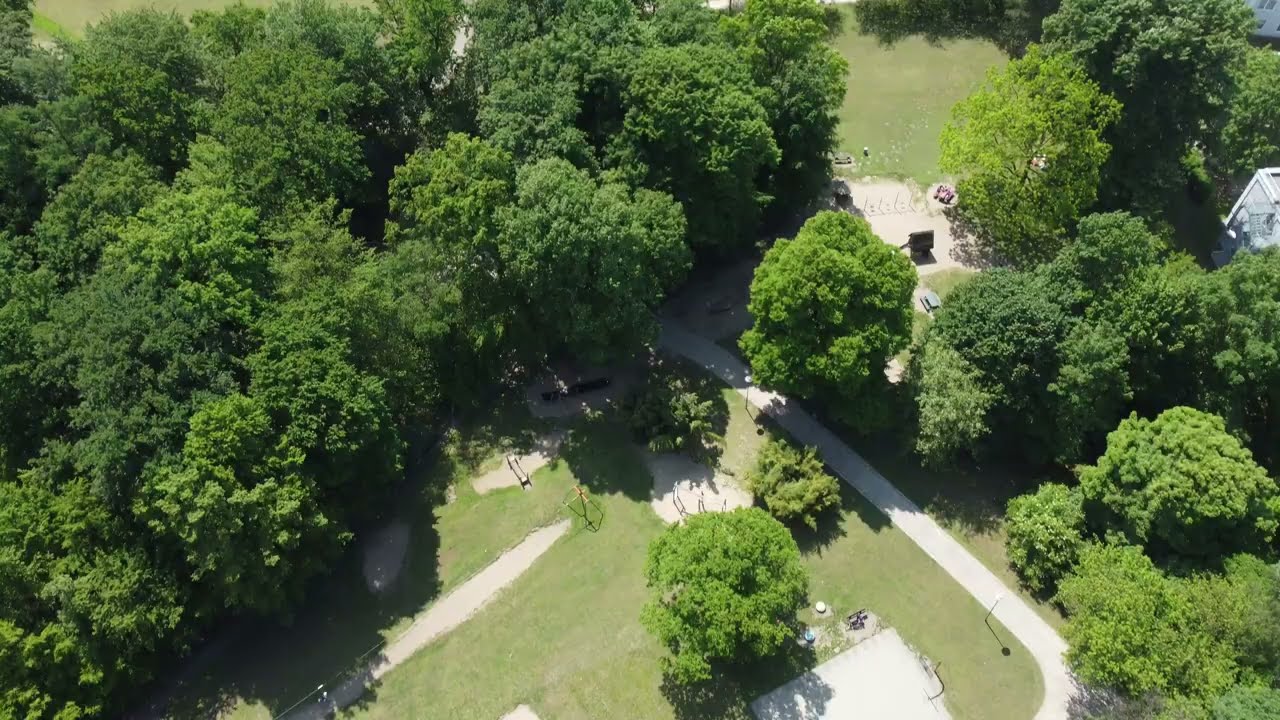This photorealistic aerial image captures a scenic park enveloped by lush, bright green trees, creating a vibrant and tranquil atmosphere. Dominating the bottom of the image, a well-maintained open field of short, verdant grass is crisscrossed by a network of white paved walking paths. Within this cleared area lies a square, gray concrete basketball court and several shady clearings housing what appear to be children's play structures. A couple of bushy green trees add to the park’s charm, providing natural shade. 

The top left portion of the image is densely populated with tall, bright green trees, while the top right hints at another grassy clearing, although details are sparse from this distance. A few white buildings are visible in the top right and bottom right corners, blending into the park's periphery. Street lights, subtle and almost hidden, cast faint shadows, indicating the daylight's source from the top left. The rest of the image showcases the dense foliage of the trees that surround and outline the cleared areas and paths, creating a harmonious blend of natural greenery and recreational space.